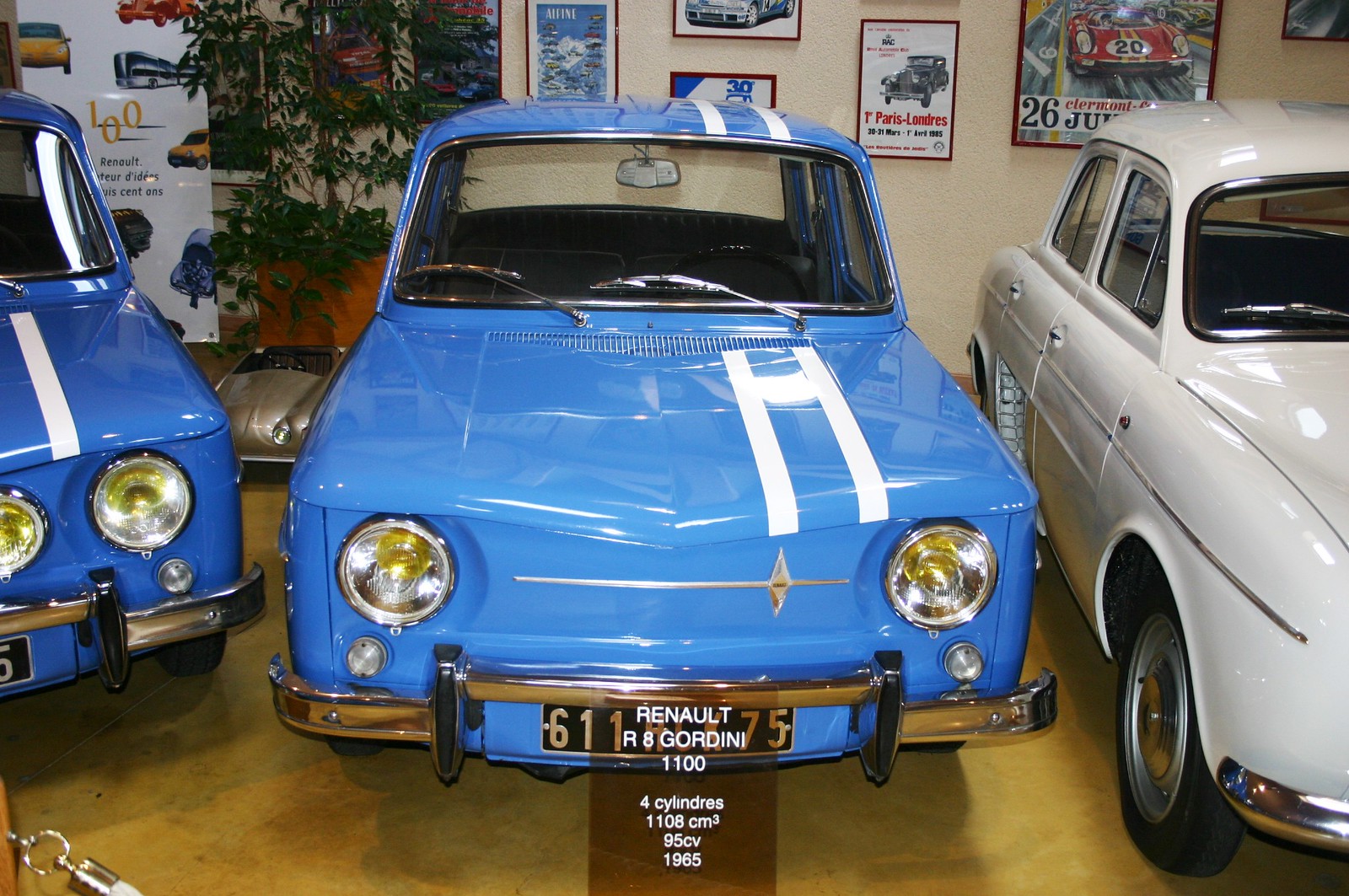The photo captures a classic car museum showroom with a distinct, warm ambiance accentuated by a tan wall and a polished yellow floor. Centerstage is a vintage blue car embellished with two parallel white racing stripes that extend from the hood to the back, identified as a Renault R8 Gordini, 1965 model with a four-cylinder 1108 cm³ engine offering 95 CV. To the left of this mid-sized, boxy sports car, partially cut off, is another vintage blue car, possibly a shade darker and older, designed with a similar classic aesthetic. On the right is an off-white car which is also partially visible. The background hosts various car photographs and placards, contributing to the museum-like atmosphere, featuring signs and text including "T Paris" and "26." Among the decor is a solitary potted plant, adding a touch of greenery to the predominantly classic, automotive-themed interior.